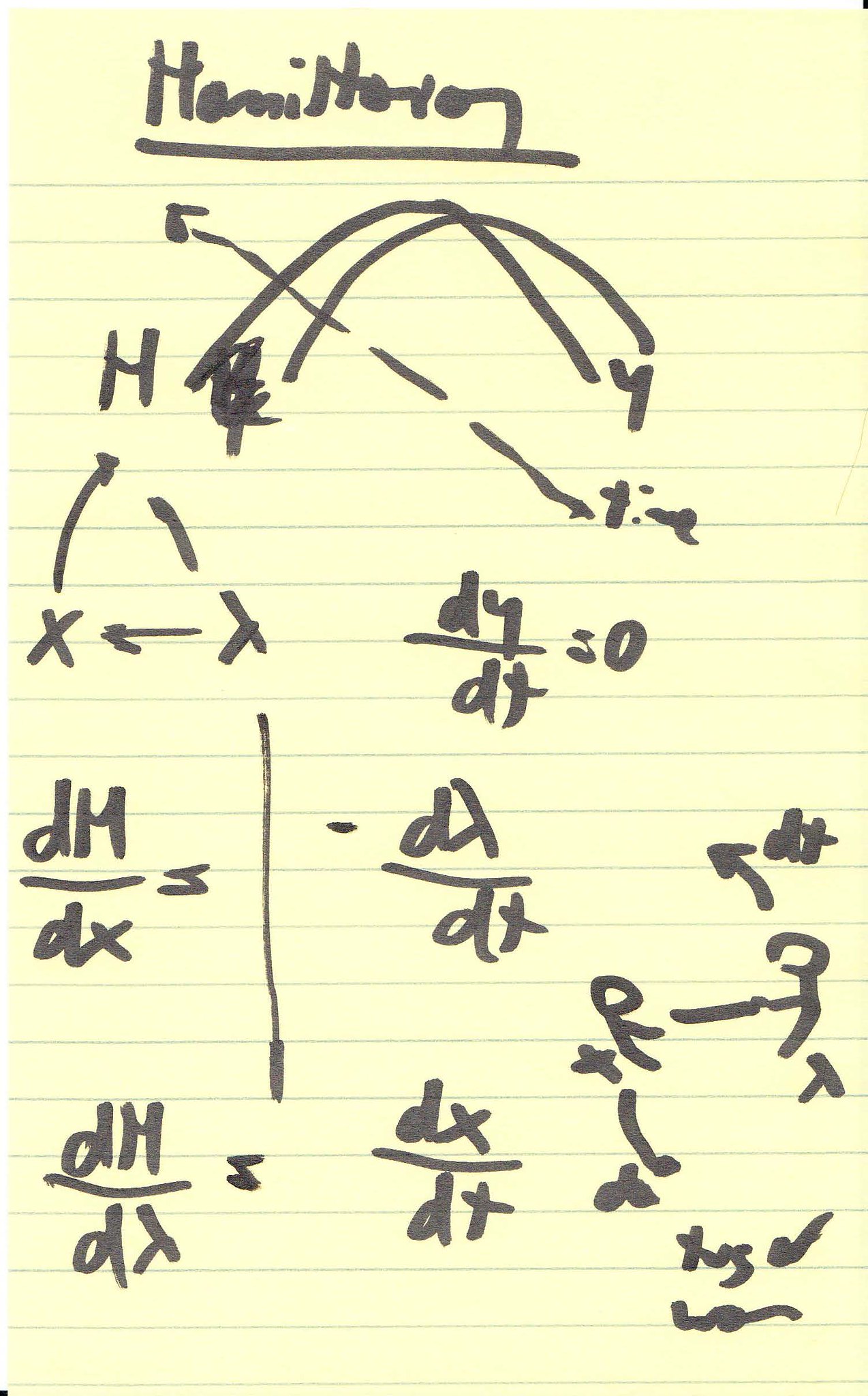This color scan showcases a piece of yellow legal pad paper, a typical lined writing paper. At the top, written in a thick, dark (nearly black) magic marker, is the word "Hamilton," which is underlined for emphasis. Beneath this bold heading is a collection of handwritten football plays, intricately sketched out. These plays, likely defensive formations, comprise a multitude of arrows — both curved and dotted — which chart out various strategies. Interspersed among the diagrammed plays are several mathematical formulas, presented as fractions and polynomials. These notes, clearly penned by hand, suggest a melding of athletic strategy and mathematical analysis. Additionally, about three-quarters down the right side of the paper, two stick figures face each other, with arrows extending from them toward the nearby polynomial fractions, possibly indicating a relationship between the figures and the mathematical expressions or strategies. The entire page is a fascinating blend of sports tactics and mathematical calculations, offering a glimpse into the mind of the note-taker.